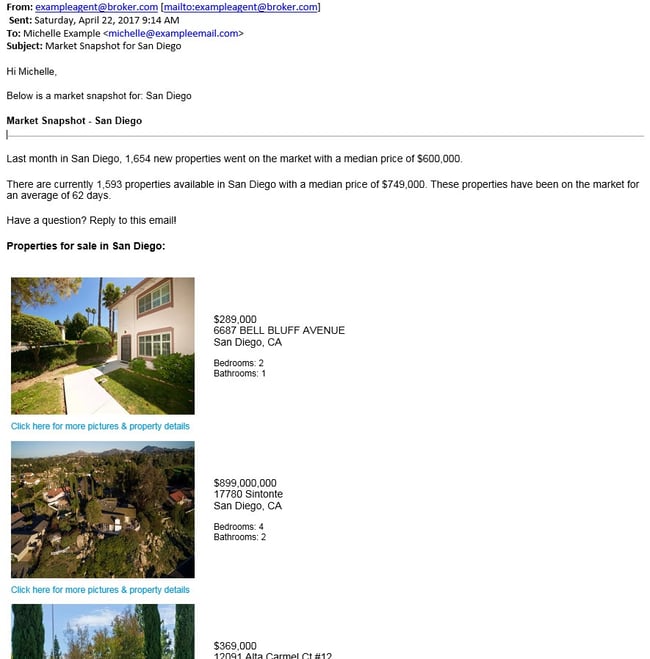The image showcases an email detailing a market snapshot for San Diego, sent on Saturday, April 22, 2017, at 9:14 AM. The email is addressed to Michelle at example.email.com from the sender example.agent@broker.com at broker.com. 

The subject of the email is "Market Snapshots for San Diego." The email begins with a greeting, followed by an overview of the real estate market in San Diego. The snapshot reveals that last month, 1,654 new properties were listed with a median price of $600,000. Currently, there are 1,593 properties available, with a median price of $749,000. These properties have been on the market for an average of 62 days. Recipients are encouraged to reply to the email with any questions.

Following the market overview, the email highlights three properties for sale in San Diego, each accompanied by images. 

- The first property, priced at $989,000, is located at 6687 Bell Bluff Avenue, San Diego, California. It features 2 bedrooms and 1 bathroom. The image shows the front entrance with a concrete walkway leading to a private yard surrounded by lush vegetation.
  
- The second property, listed for $899,000, is situated at 17780 Senda Encantada, San Diego, California. It includes 4 bedrooms and 2 bathrooms. The image is an aerial view of the home, indicating it is located in a wooded area with some acreage, providing a sense of privacy with tree tops visible from above.
  
- The third property, priced at $369,000, is found at 12091 Alta Carmel Court #12, San Diego, California. It does not specify the number of bedrooms or bathrooms.

A link for more pictures and property details is provided beside each listing.